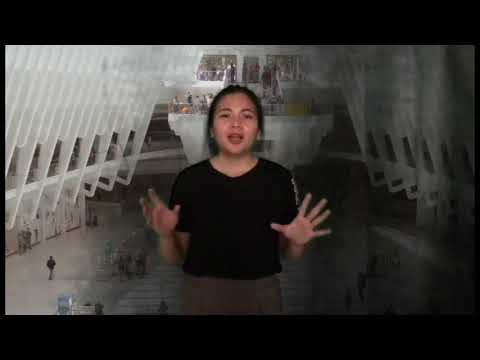The image depicts a light-skinned woman with short black hair, dressed in a black t-shirt and dark tan or brown skirt, standing in the center of a vast, dimly-lit indoor area. She is likely giving a presentation or speech, as suggested by her wide open mouth and her hands raised to chest level, palms forward with fingers splayed. The scene is framed by thin black rectangular bars at the top and bottom, giving it a letterbox appearance. Behind her, a grand atrium-like space extends, adorned with tall white beams or pillars that have a glass-like quality. This space resembles a large public hub, possibly an airport or a fancy train station, given the wide walkways and seating arrangements visible below. People are scattered on either side of the walkway, with more concentrated on the left. In the distance, there is another elevated area, resembling a balcony with people standing on it, adding to the sense of a large, open environment. Despite the grandeur of the setting, the image quality is low, appearing grainy and highly compressed.